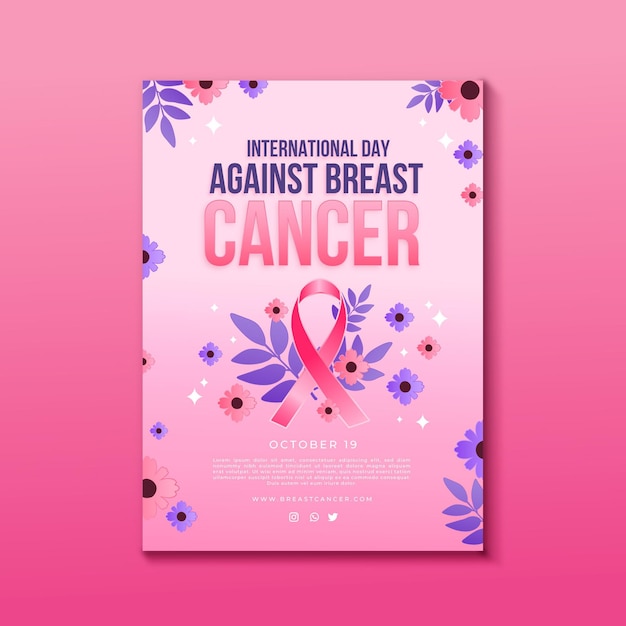The image is a detailed poster designed to commemorate the International Day Against Breast Cancer. The background presents a visually appealing gradient, transitioning smoothly from a light pink at the top to a deeper pink hue at the bottom. Centrally placed, the bold text "International Day Against Breast Cancer" commands attention. Beneath this title, a prominent pink twisted ribbon, universally recognized as the symbol for breast cancer awareness, is displayed. Further down, the date "October 19th" is clearly written in white text. The bottom portion of the poster contains what appears to be a paragraph of information, though the text is unreadable.